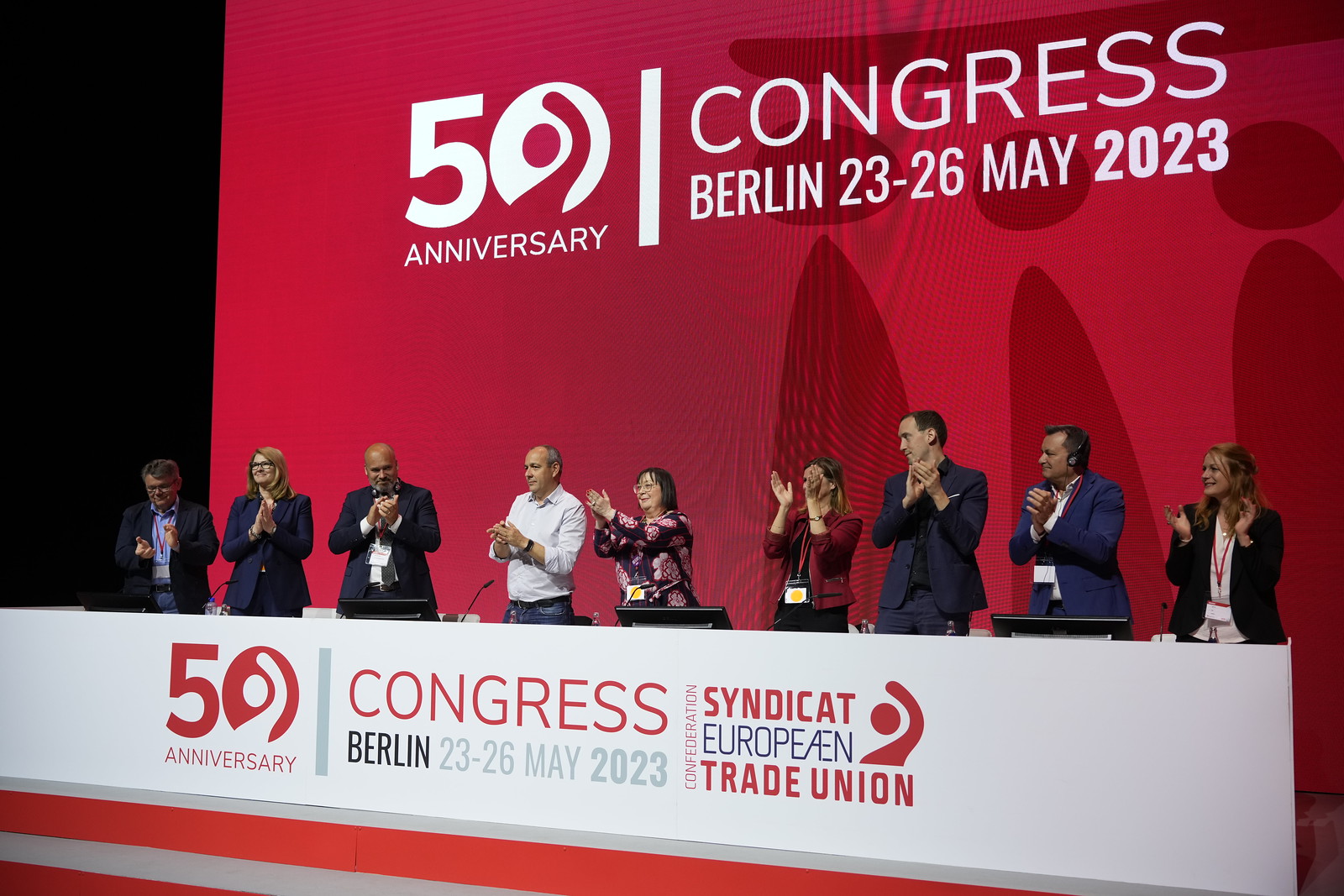This photograph captures a scene from the 50th Anniversary Congress of the European Trade Union in Berlin, held from May 23 to May 26, 2023. A total of nine people are lined up on stage, applauding. The group includes a man, a woman, two more men, two women, another two men, and one more woman. Behind them, a large red board prominently displays the event details in white font: "50th Anniversary Congress Berlin, 23 to 26 May 2023." In front of the people on stage, there are four computer monitors, likely used for reading or displaying information. A table with white fronting also bears the same event details and the text "Syndicate European Trade Union," along with a small graphic of a person. The overall color scheme includes shades of red, white, blue, tan, beige, brown, and black.